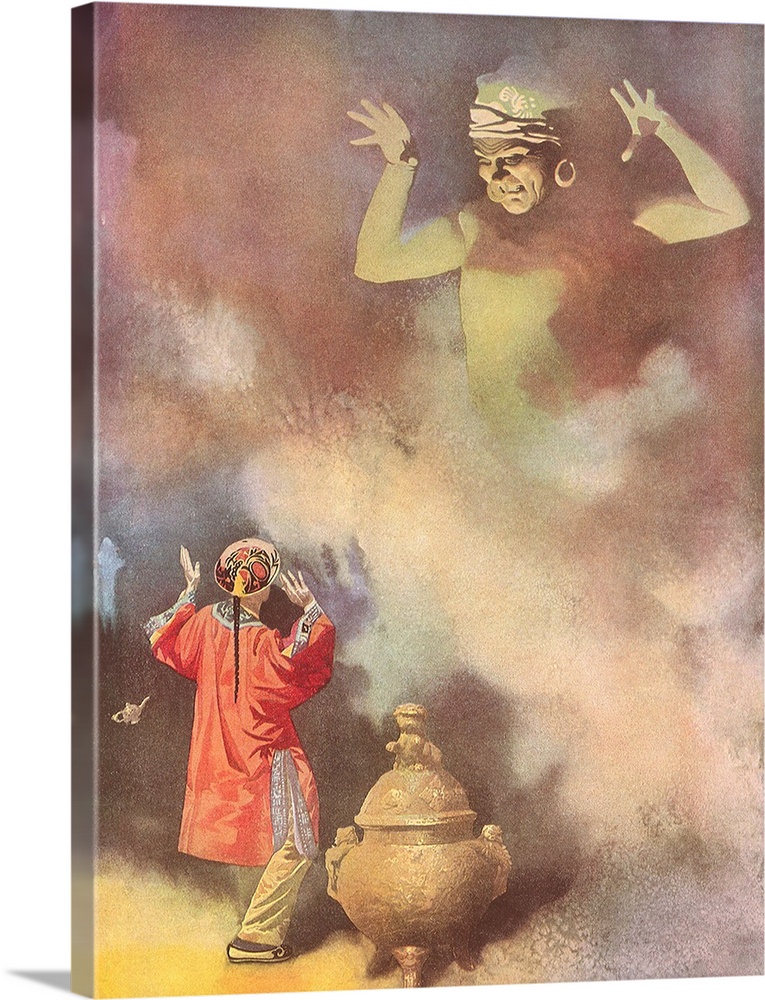The image is a vibrant, colored illustration likely on a canvas, which is noticeably thick, as indicated by the visible edge along the left border. The canvas is slightly tilted, with the left side closer to the viewer. The scene appears to depict a moment reminiscent of Aladdin releasing a genie from a lamp.

In the top right corner, a menacing genie emerges from a large stone container adorned with a foo dog, surrounded by a billowing plume of smoke that obscures its lower body. The genie, clad in a white tall turban with gold hoop earrings, has both arms raised with fingers spread out in a claw-like manner. The genie sports a dramatic expression that could be interpreted as either smiling or menacing.

Positioned in the bottom left corner, there is a person who seems startled, leaning back with their arms raised in a similar pose to the genie. This individual, possibly of Chinese descent, is depicted with a round hat, black hair in a single long braid, and dressed in a detailed, flowing orange robe over light brown pants and slippers. The intricate depiction captures the ripples and texture of the robe, emphasizing the character's dynamic reaction.

To the immediate right of this person, partly suspended in mid-air, is a large rounded lamp, its top featuring a small animal or perhaps a figurine. This lamp is situated closer to the viewer, serving as the pivotal element from which the smoke and the genie emerge. The combination of these elements— the detailed characters, the dramatic smoke, and the mystic lamp— crafts a vivid and intricate scene.